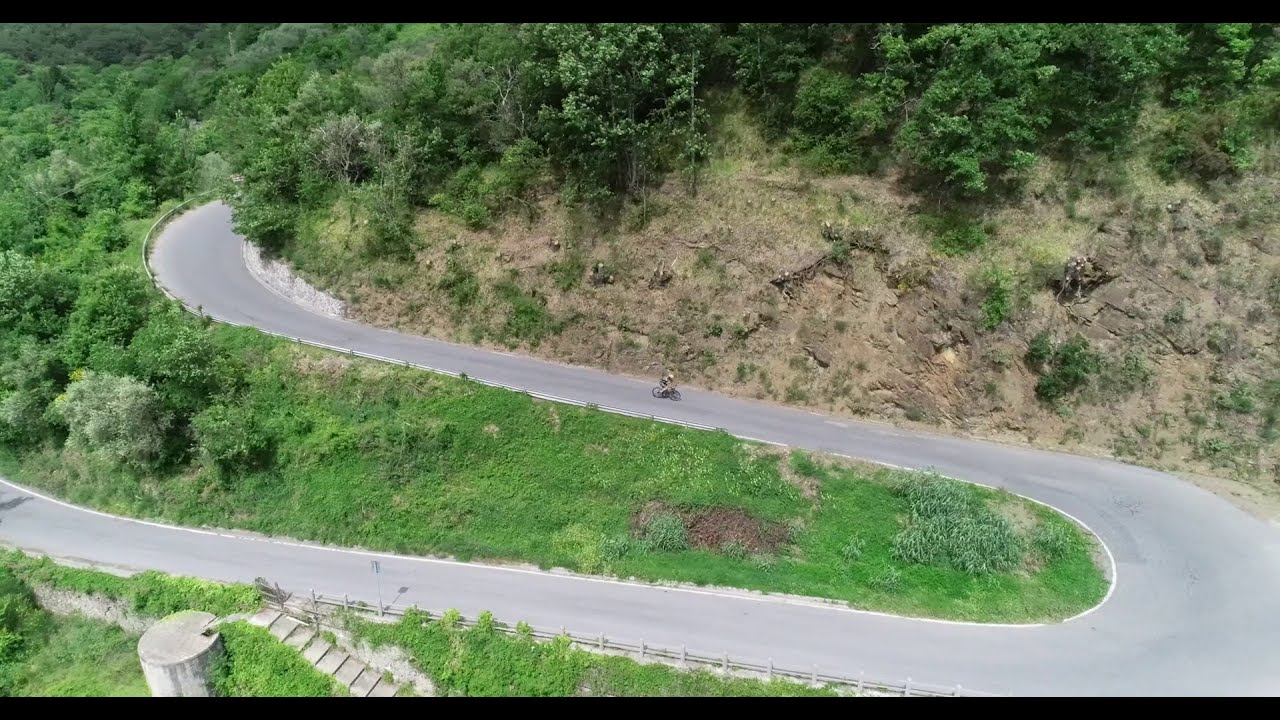This detailed color photograph, taken from an aerial drone view and presented in landscape orientation, captures a winding mountain road that snakes through lush, green hillsides in a distinct S-shape. The narrow image, bordered by horizontal black bars at the top and bottom, showcases a roadway that extends from the bottom right corner, curves dramatically to the left and then back to the right, disappearing behind the verdant landscape. Along the upper bend, a lone bicyclist or moped rider, too distant to identify clearly, navigates the curves. The scene is framed by a rocky cliff face crowned with thick, bushy trees, and the spaces between the bends are filled with dense green grass and brush. In the bottom left corner, a concrete storage tank is accessible by a small stairway descending from the road, though its destination remains unseen. The dirt embankment to the top right adds texture to the picturesque setting, enhancing the representational realism of the photograph.